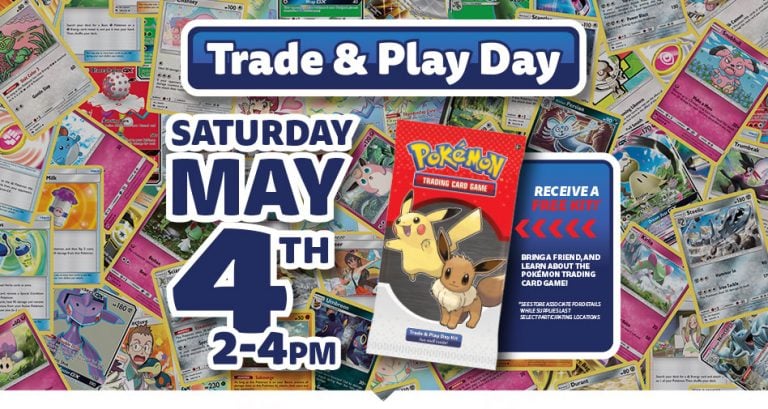In this vibrant and engaging image, the central visual element is a rectangular box positioned at the top middle, boldly displaying the words "Trade and Play Day" in a thick, large white font. The box's background is a striking bluish hue, while its borders are neatly outlined in white. Just below this, on the left side, are the details for the event: "Saturday, May 4th, 2-4pm," presented in a matching dark blue font with white borders.

On the right side of the image, a Pokemon card pack prominently features the iconic Pokemon logo at its top, characterized by a yellow interior and a blue outline. The card pack showcases images of Pikachu and Eevee. The overall background of the image is a dynamic spread of various Pokemon cards scattered across the floor, with a notably pink card visible at the top right.

Centrally placed beside the Pokemon pack is a square-shaped highlight, containing the text "Receive a Free Kit." The phrase "Receive A" is in white, while "Free Kit" is accentuated in red. Surrounding this text are five arrows pointing left towards the pack. Below this square, the invitation "Bring a friend and learn more about the Pokemon Trading Card Game" encourages participation and social engagement.